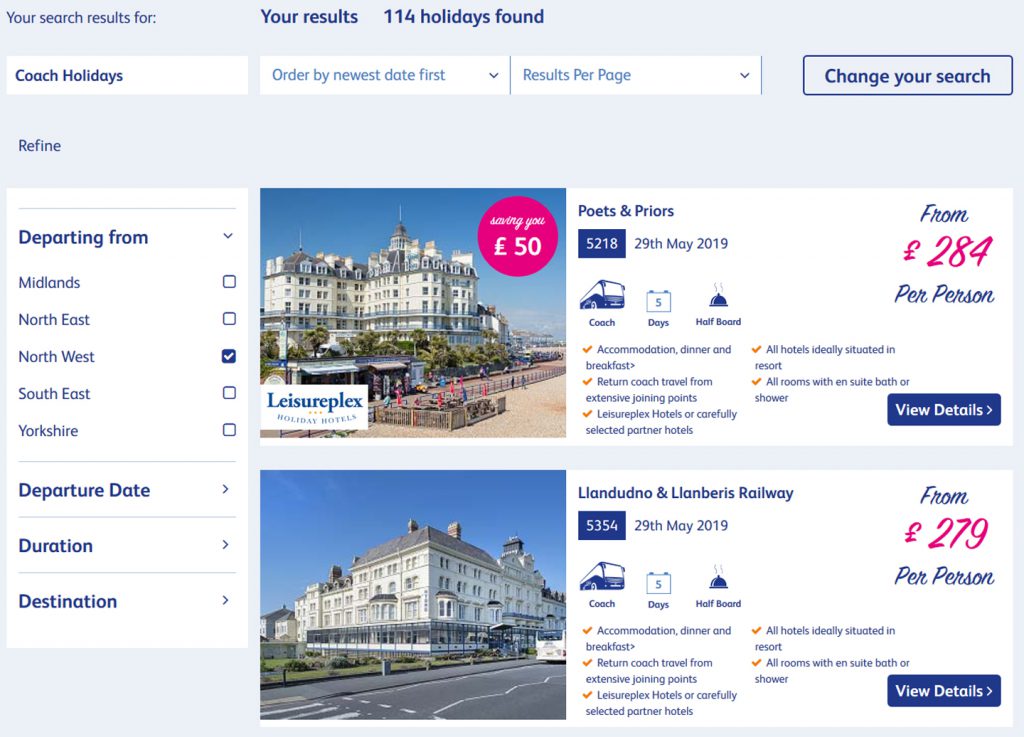**Detailed Description of Railway Options for Coach Holidays on May 29, 2019**

This screenshot showcases the search results for "Coach Holidays" on a travel booking website, specifically ordered by newest entries. The user has opted for multiple results per page and has a particular interest in destinations located in the northwest of a designated area.

1. **Option 1: Poets and Priors**
   - **Date:** May 29, 2019
   - **Price:** £284 per person
   - **Package Details:**
     - **Travel:** Return coach travel from extensive joining points
     - **Accommodation:** Stay at Leisureplex hotels or carefully selected partner hotels, all ideally situated within a resort.
     - **Amenities:** All rooms feature en-suite bathrooms with either a bath or shower.
     - **Inclusions:** Accommodation includes dinner and breakfast.
     - **Additional Highlights:** The package offers a comprehensive experience with coach rides and well-appointed lodging.

2. **Option 2: London Dunno and Lone Barris Railway**
   - **Date:** May 29, 2019
   - **Price:** £279 per person
   - **Visuals:** Accompanied by a picture of a large white building adorned with many windows.
   - **Package Details:**
     - **Travel:** Return coach travel from extensive joining points.
     - **Accommodation:** Stay at Leisureplex hotels or other carefully selected partner hotels, all ideally located within a resort.
     - **Amenities:** All rooms come with en-suite bathrooms equipped with either a bath or shower.
     - **Inclusions:** Accommodation includes dinner and breakfast.
     - **Additional Highlights:** Similar to the first option, this package provides a well-rounded travel experience with comfortable lodging and comprehensive meal plans.

Both options offer excellent value and convenience, featuring well-located and comfortable accommodations along with inclusive meal services, ensuring a delightful coach holiday experience.